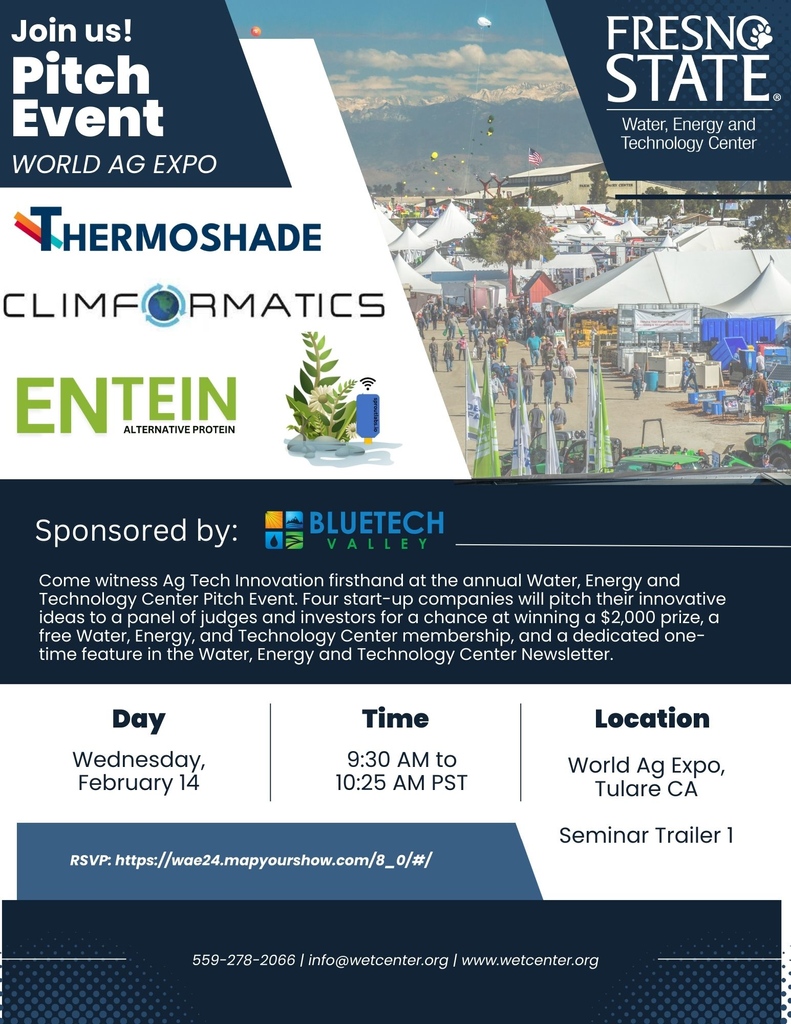Join us at the World AG Expo in Tulare, California on Wednesday, February 14th for the Water Energy and Technology Center's Pitch Event. The event will feature innovative presentations from four startup companies: Thermoshade, Climaformatics, and Intine Alternative Protein. Set against a scenic outdoor backdrop with white tents and attendees, this event promises an exciting showcase of AG tech innovations. Sponsored by BlueTech Valley, the pitch event will see these startups competing for a $2,000 prize, a free membership at the Water Energy and Technology Center, and a one-time feature in its newsletter. The details are displayed prominently in the poster: from 9 a.m. to 10:25 a.m. PST, with the sponsorship of Fresno State Water Energy and Technology Center highlighted at the top right. Don't miss this opportunity to witness cutting-edge technology in agriculture.